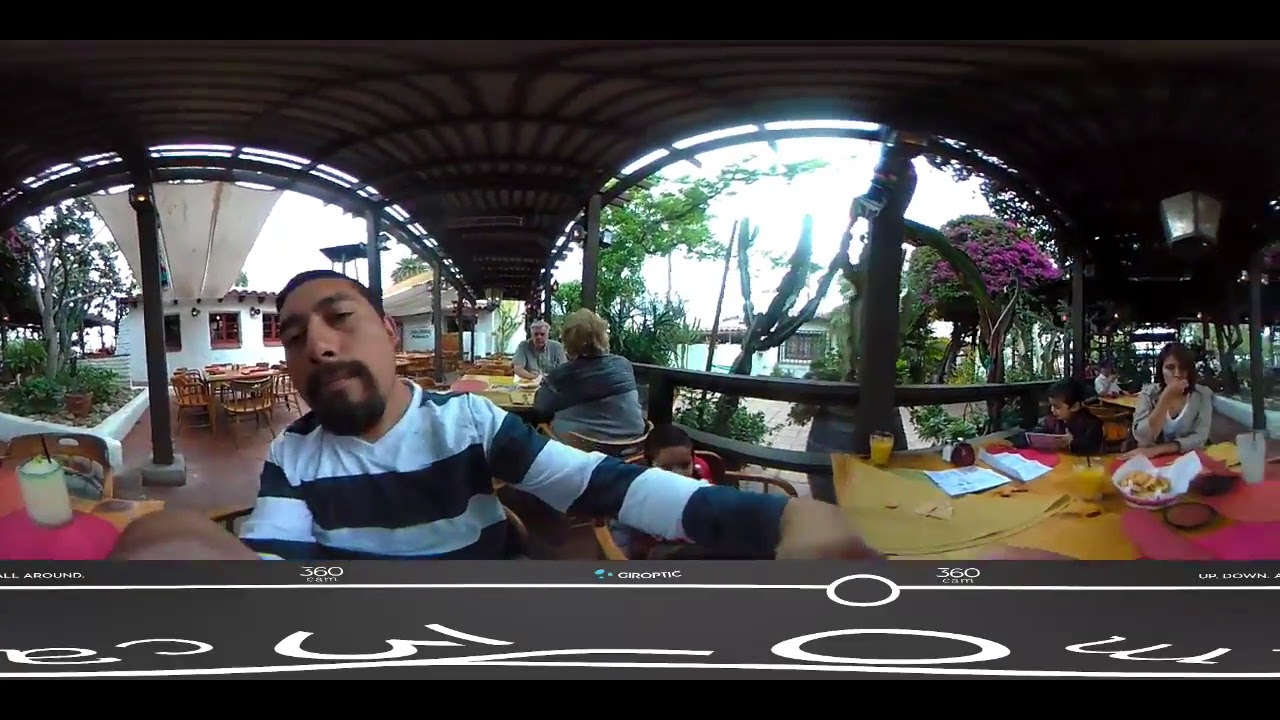In this horizontally aligned rectangular image, the scene is set in an open-air restaurant with a metal roof, structured with two arches leading to other outdoor sections. The backdrop reveals a bright white sky dotted with trees, including one with vibrant purple flowers. The foreground prominently features a man with very short black hair and a brown goatee, wearing a navy-blue and white striped T-shirt. His hand extends forward, possibly taking the picture. 

To the right, a woman and a child are seated at a table covered with brown papers and a basket of food. The child, who appears to be holding a menu or an iPad, has an orange juice in front of them, while there is a drink in front of the woman, who rests her elbow on the table and her hand over her mouth. Beside them sits another table with two elderly couples: an older man with white hair and a woman with short light brown hair, whose backside is visible.

In the lower part of the image, there is a thick gray border decorated with white symbols and letters, including the number 360 and the word "gyro." The overall setting is outdoor and warm, with multiple colors like black, brown, tan, white, green, pink, purple, orange, yellow, and gray visible throughout the image, enhancing the vibrant, tropical atmosphere of the restaurant.